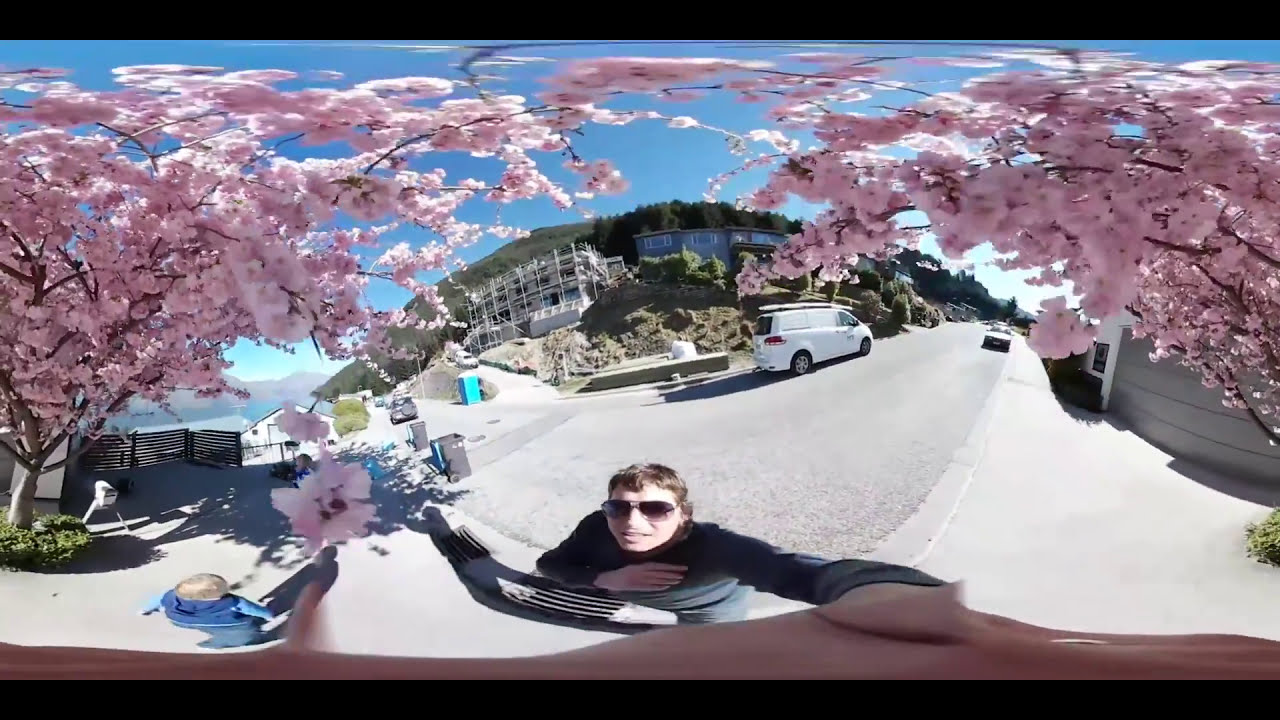In this horizontally aligned image framed by black borders on the top and bottom, a man takes a selfie from an upper angle. He stands centrally at the bottom of the image, looking up towards the camera, wearing brown sunglasses and a black long-sleeve shirt. He has short brown hair. Beside him in the lower left corner, there's another person with blonde hair wearing a blue vest over a lighter blue long-sleeve shirt. The background reveals a clear blue sky and a picturesque neighborhood scene. On both sides of the man, trees with pink and light purple flowers extend over the road, mingling at the top center of the image. In the distance, a large multi-story white building, possibly a condominium, and a gray building with a brown roof are perched on a hill surrounded by tall trees. A street runs behind the man, where a white van drives to the right, with another car coming from the opposite direction. The vibrant colors and outdoor setting suggest it's taken during the middle of a sunny day.